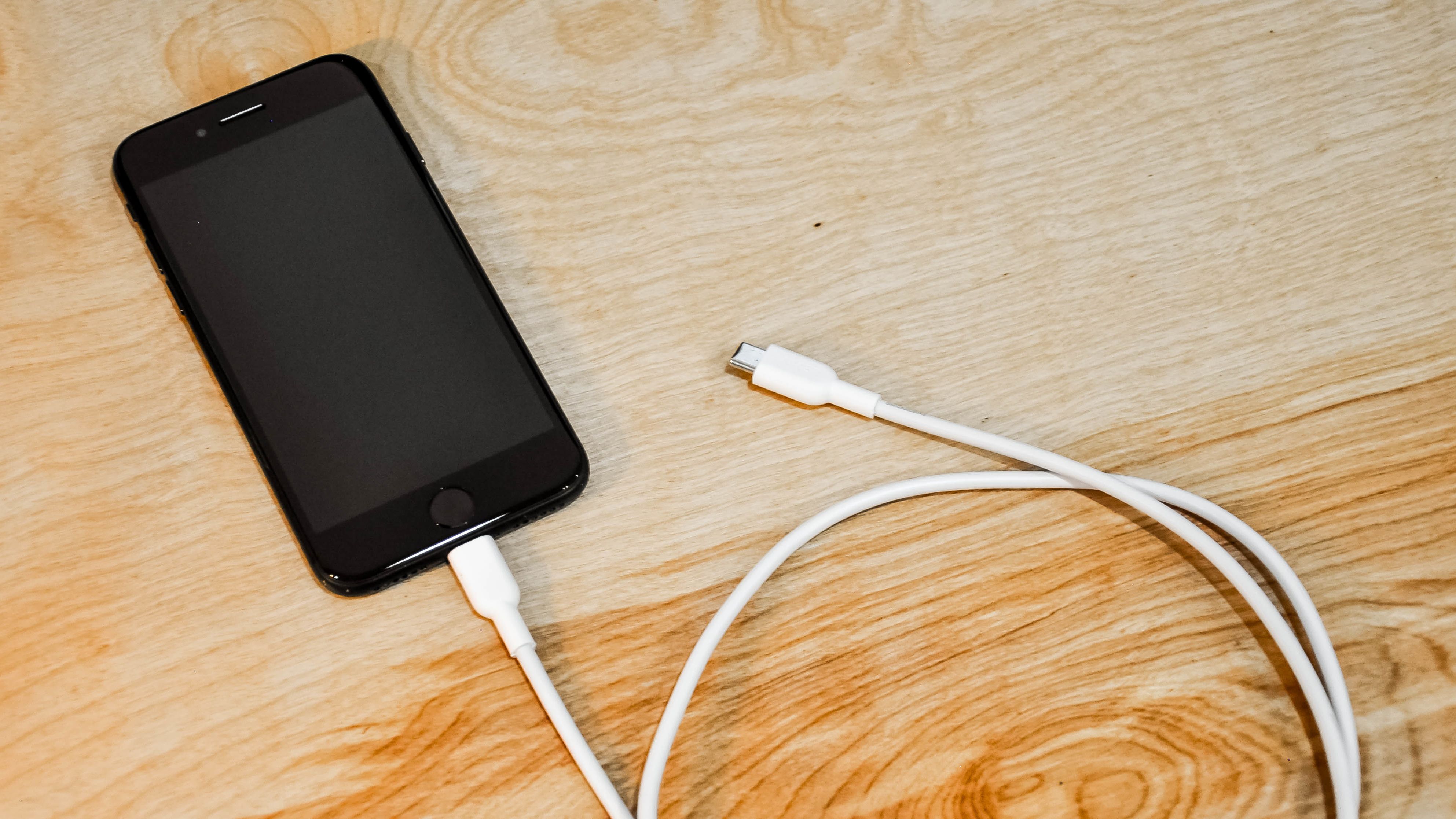The image shows a close-up, top-down view of an older model black iPhone lying on a wooden table. The phone, which features a circular home button and buttons on the top edge, is positioned in the upper left corner of the image. The wooden table's color gradient shifts from a light tan near the top to a darker brown towards the bottom. The iPhone, which has its screen turned off, is connected to a white, coiled charging cable. The cable stretches from the bottom of the phone towards the right side of the picture, with the loose end resting unconnected on the table, featuring a small silver metal connector.